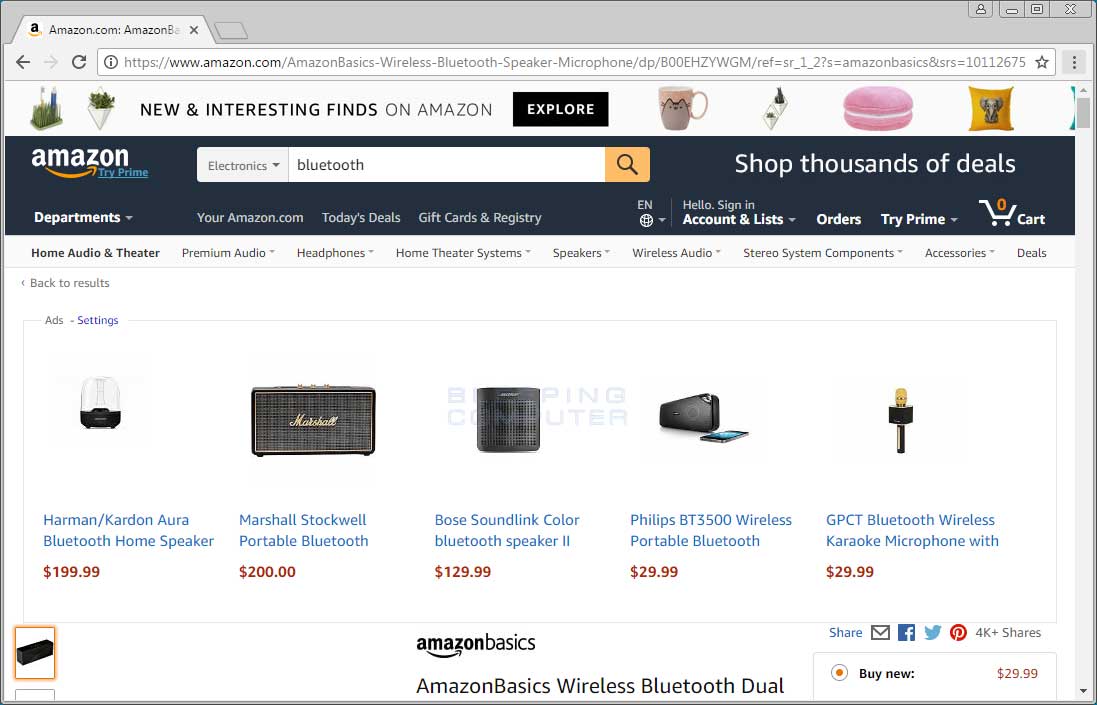The image depicts the Amazon website search page, specifically for the term "Bluetooth." In the upper left corner, the browser tab displays "Amazon.com," though some details are cut off. Directly below, there is a left arrow and a gray right arrow, alongside a refresh arrow. 

In the address bar, the URL for the search page is visible. Below it, on the left, are two icons; one resembles a plant and is labeled "New and Interesting Finds on Amazon." To the right, a long black box labeled "Explore" is present, followed by four small media images representing products, such as a coffee cup with a design. 

Further down, on the left, a section labeled "Amazon TryPrime" appears with a search area below it. This section includes a drop-down menu labeled "Electronics," with the search term "Bluetooth" and a magnifying glass icon. Adjacent to this, a promotional banner reads "Shop Thousands of Deals."

Beneath the promotional banner, on the left side, a drop-down menu labeled "Departments" is visible. To the right, there are links for "Today's Deals," "Gift Cards," "Registry," "Hello, Sign in," "Accounts & Lists," "Orders," "TryPrime," and a shopping cart icon showing zero items. Additionally, product listings with item names and prices are visible, accompanied by social media icons at the bottom of the page.